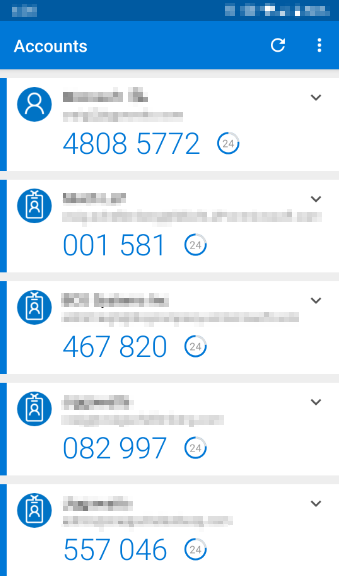This screenshot appears to be from a mobile device, with significant portions of the interface pixelated for privacy. At the top, the usual status icons, including the battery meter, are obscured. Below this, a light-colored navigation bar displays the header "accounts" on the left, a refresh button in the center, and a three-vertical-dot menu on the right. Following this bar, five sections are distinguished by vertical blue lines along the left edge.

Each section contains a mix of icons and text, although most personal details are pixelated. In the first section, an icon of a person—displaying a head and shoulders in blue—precedes the phone number "4808 5772." On the far right of this section, there is an option for a dropdown menu.

The subsequent four sections feature a different icon: a profile picture framed by what appears to be a lanyard. The associated phone numbers for these sections are as follows:
- "001-581"
- "467-820"
- "082-997"
- "557-046"

Each phone number section includes a circle with the number “24” inside it, in gray. The top right quarter of this circle is gray, while the remaining three-quarters are blue.

Overall, the key elements within this screenshot are identifiable despite the significant pixelation intended to preserve privacy.